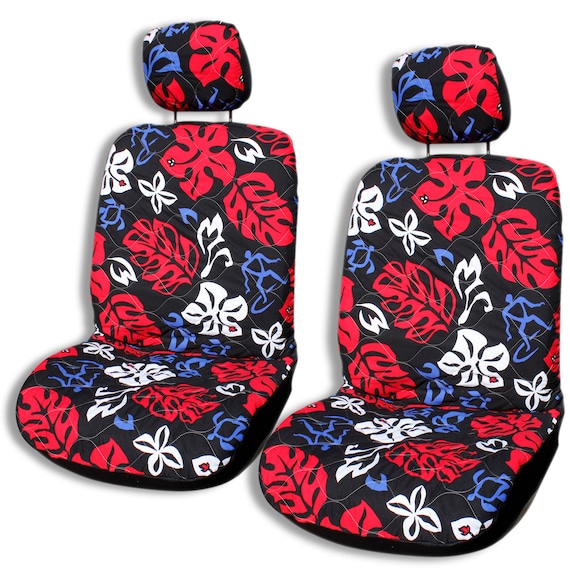The image features two car seats adorned with custom covers. The seat covers exhibit a Hawaiian-themed design with a black background. They are detailed with vibrant, tropical floral illustrations, including red and white hibiscus flowers, some of which have five petals, others four. The design also includes red leaves, blue turtles, and a blue stick figure on a surfboard, accentuating the tropical motif. The covers are already installed on the seats, showing sections that attach to the lower part and the headrests, which are elevated by two metal bars. The seats are depicted at an angle, facing slightly toward the bottom left of the image.